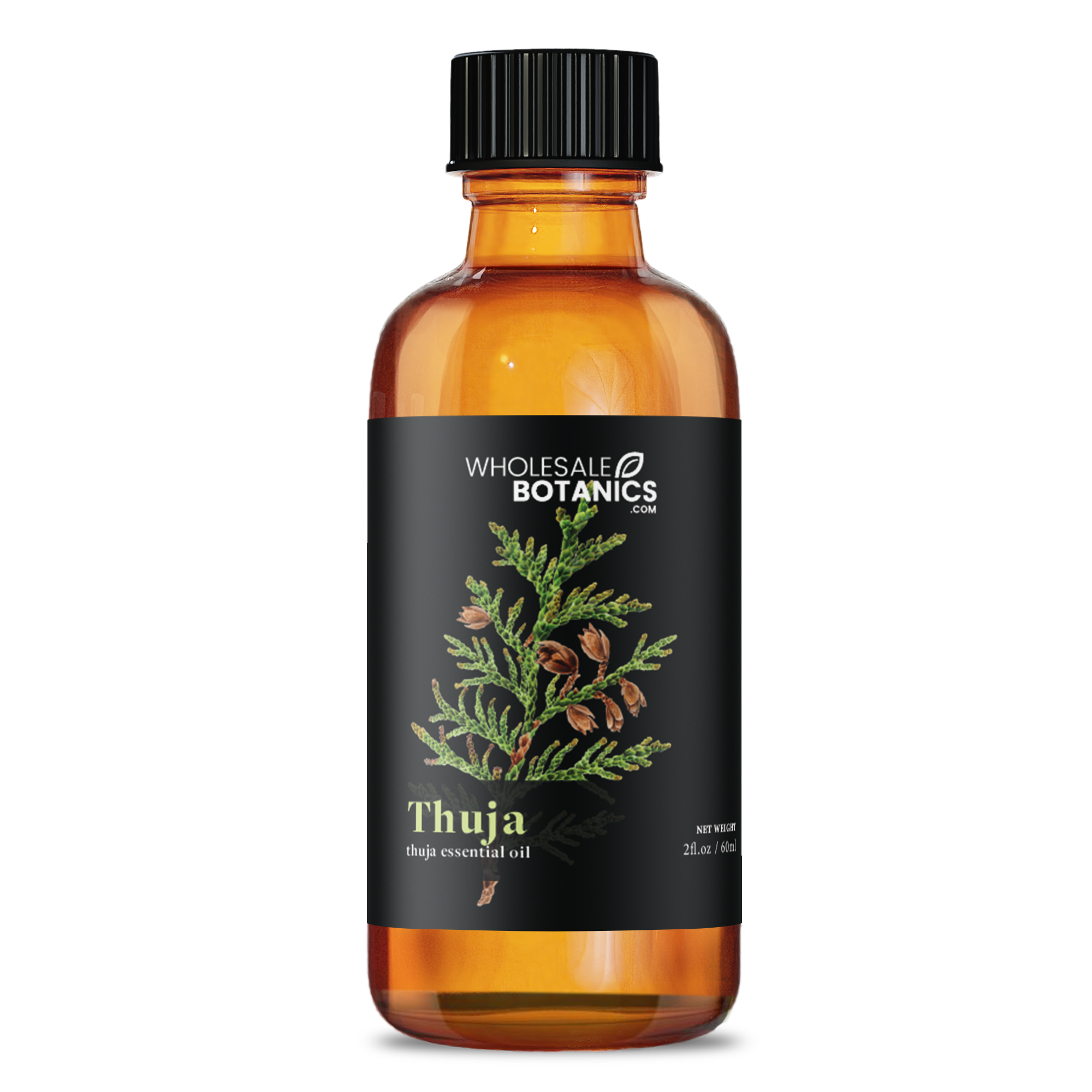This image depicts a product photo of a Thuja essential oil bottle from Wholesale Botanics, set against a pure white background, enhancing its advertisement appeal. The bottle, crafted from amber-colored glass, features a sleek black cap. Its label is notably black, detailing "wholesalebotanics.com" in white and prominently showcasing Thuja essential oil in a vivid green font. The label also includes a botanical illustration resembling a herbal leaf with brownish-purple offshoots, reminiscent of a Christmas tree branch. The bottom of the label specifies the volume as 2.2 fluid ounces, making this a compact yet elegant-looking bottle.